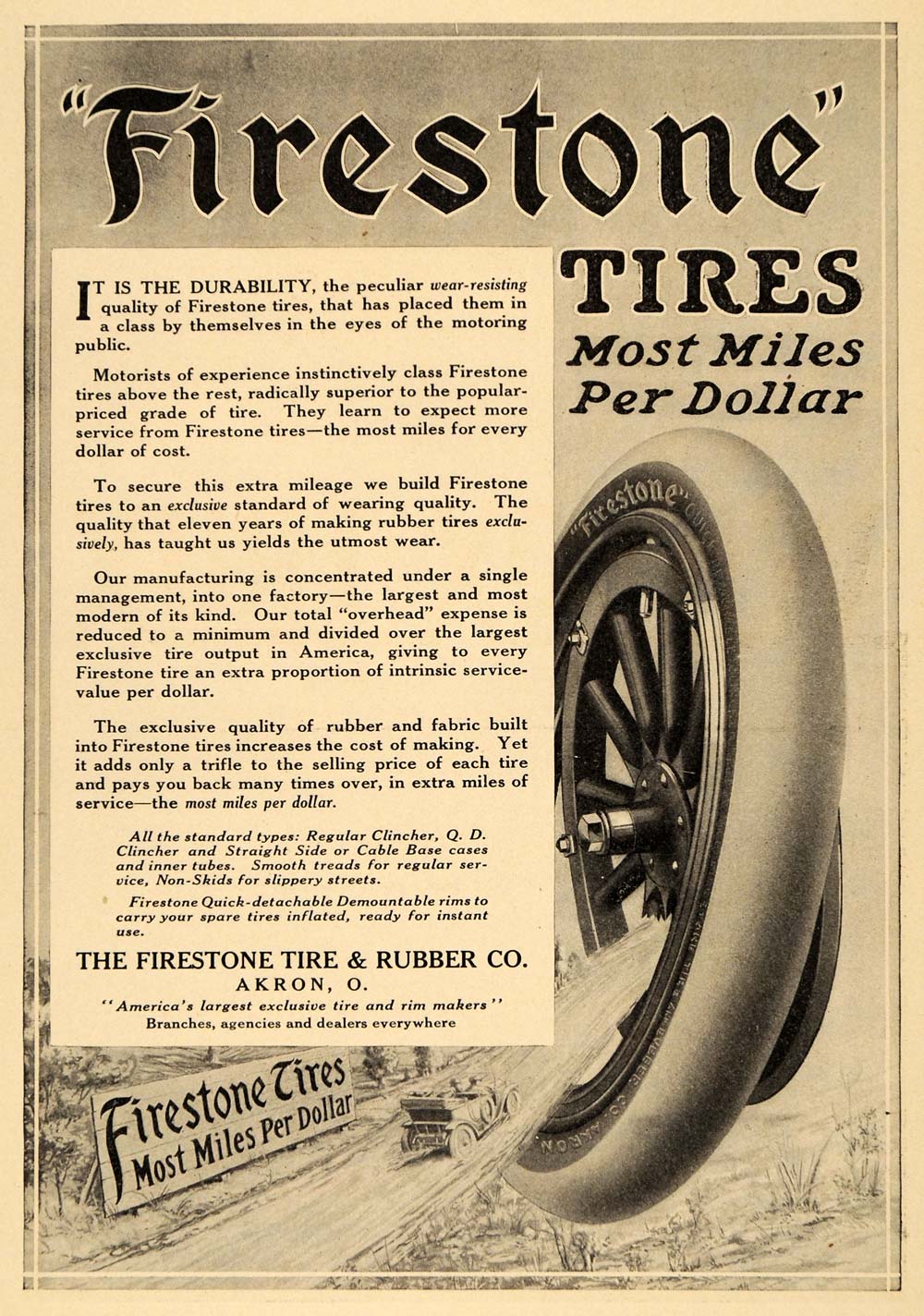This vintage black and white Firestone tires advertisement, now yellowed with age and bearing a slight sepia or pink tinge, showcases the early 1900s craftsmanship of its time. The top of the ad prominently features the phrase "Firestone tires, most miles per dollar" in a bold Times New Roman font with quotation marks. On the right side, a large, old-style tire is illustrated, looking almost like a thick bicycle tire with visible individual spokes and the Firestone brand marked in black on its white surface. 

A rural highway scene is depicted beneath, with an antique car traveling along a sketch-like dirt road that leads directly into the giant tire. A roadside sign along this road reiterates the slogan, "Firestone tires, most miles per dollar." To the left, a detailed text praises the durability and superior wear-resistance that distinguishes Firestone tires, emphasizing their extensive mileage and cost-efficiency. The advertisement claims Firestone’s manufacturing excellence, honed through eleven years of exclusive tire production, and highlights their extensive manufacturing capabilities centralized in Akron, Ohio, recognized as America's largest exclusive tire and rim makers. The ad concludes with a note on the range of available Firestone tire types and the company's widespread distribution through branches, agencies, and dealers nationwide.